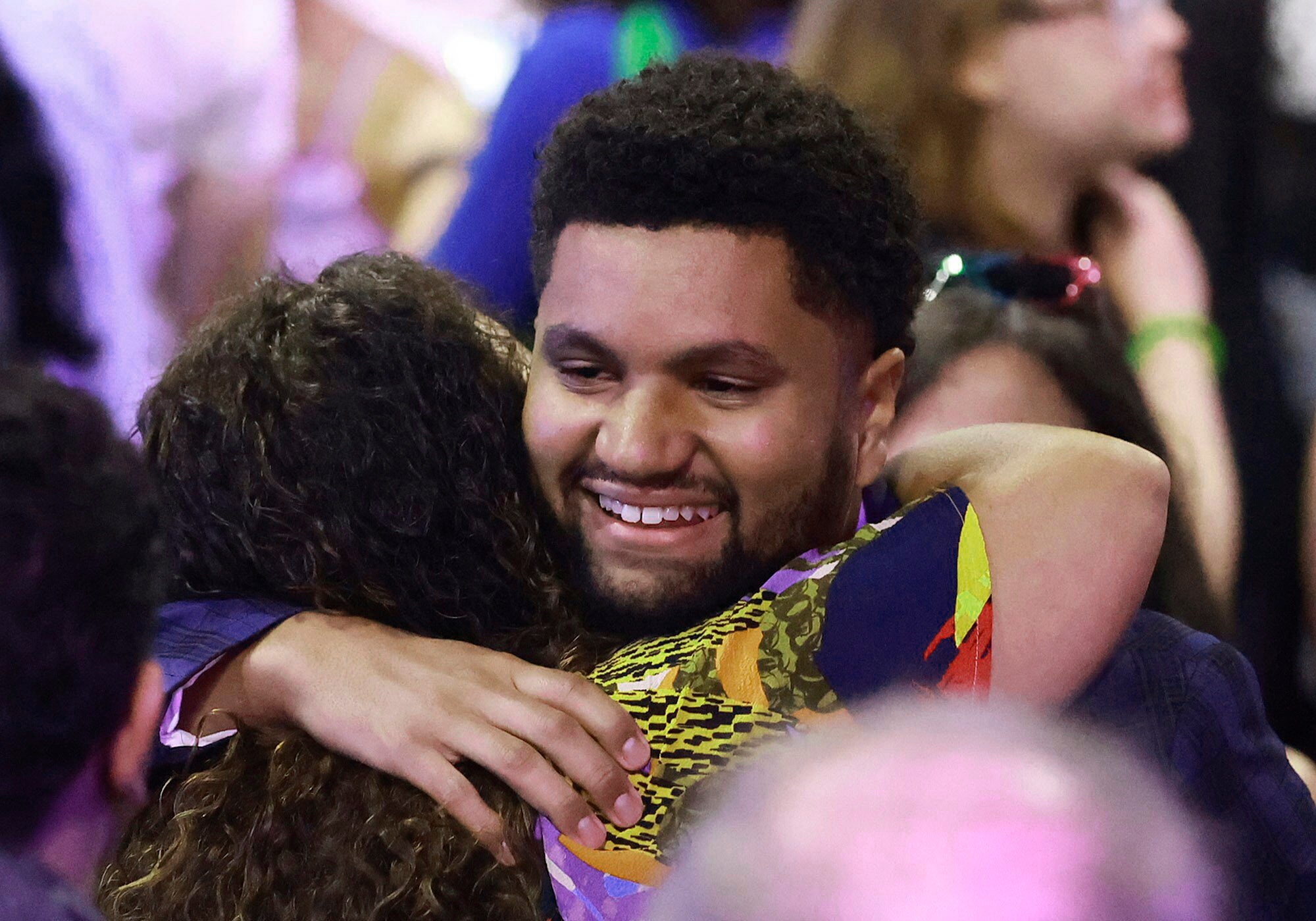This photograph captures an intimate moment between a man and a woman hugging, standing out in sharp focus amidst a blurred crowd, suggesting a larger gathering. The man, with a brownish, medium skin tone, short afro, and curly black hair, is smiling warmly, revealing white teeth. He has a short, curly black beard and a mustache, and his right hand is visible behind the woman's back. The woman's face is obscured as she is turned towards him, but she has long, thick, wavy black hair. She is wearing a vividly multicolored outfit with patterns in green, red, purple, orange, yellow, and black. In the background, although out of focus, other people are standing around, including a woman with sunglasses perched on her head, featuring blue and red frames.